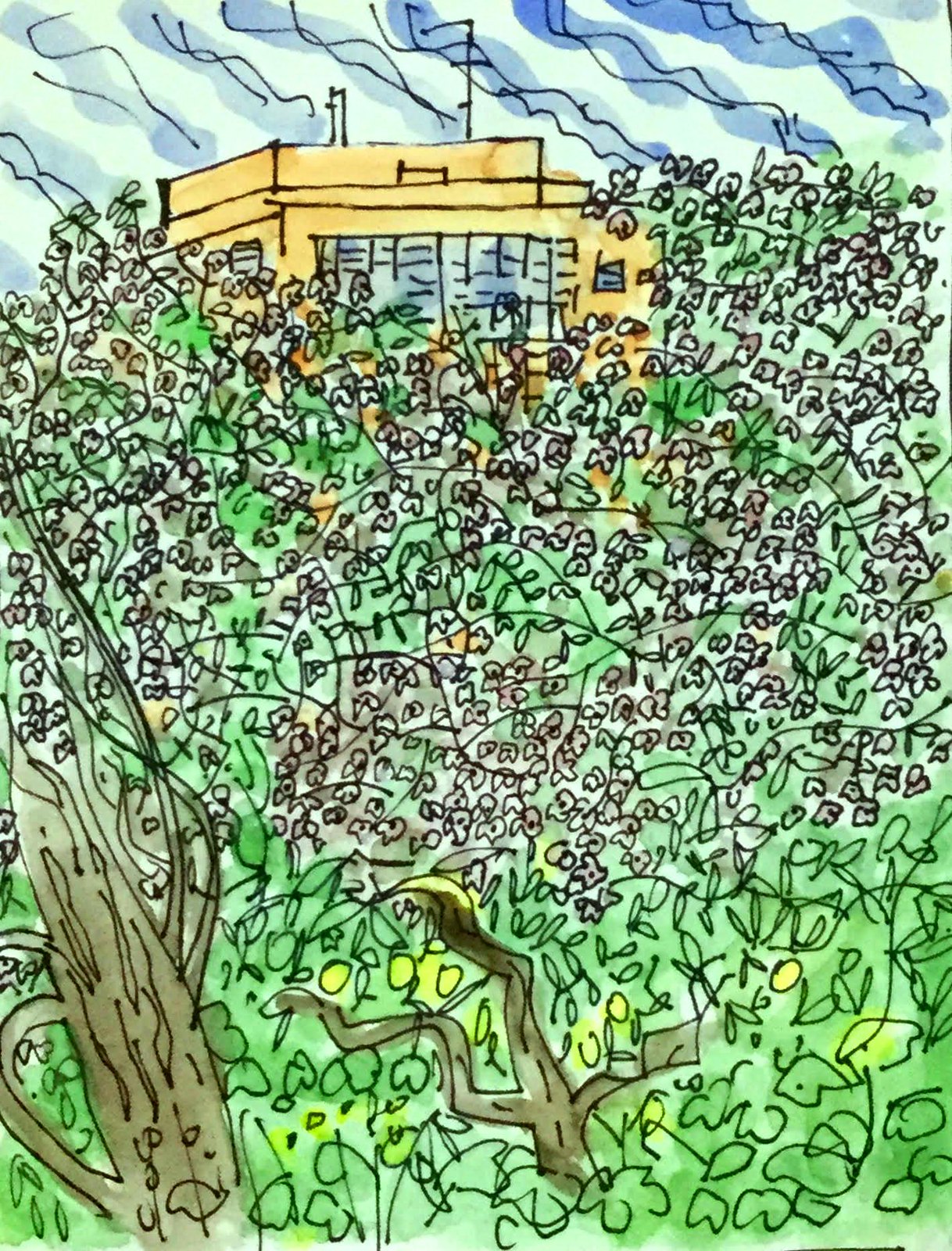The image is a detailed sketch featuring a blend of pen outlines and watercolor painting. At the center of the artwork, there is a large building characterized by a yellow or pale beige color, with noticeable big glass windows and a flat roof topped with an antenna. The building's lower part is partially obscured by lush foliage and several tree trunks painted in brown. These trees, which dominate the foreground, are adorned with green leaves, numerous pink flowers, and a scattering of round, yellow fruits. The background showcases a landscape that appears to be a verdant hill or field, depicted with varying shades of green and pale yellow, suggesting grassy terrain with occasional flowers. Above the scene, the sky is vividly rendered in a gradation of blue hues, featuring wavy and squiggly lines that imply the presence of clouds. The overall style of the image is distinctly hand-drawn, combining the precision of pen outlines with the soft, textured quality of watercolor.